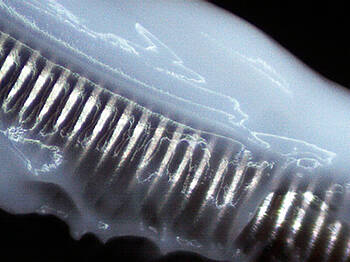This is a close-up photograph featuring a mysterious metal object that closely resembles a series of disk-like threads, possibly a screw or bolt, encased in a semi-opaque white substance. This substance, which might be ice, plastic, or a glue-like goop, envelops the metal object, appearing more opaque on the sides while remaining transparent in the middle. The encasement of the metal object seems haphazard, as if it melted around the grooves and then solidified, but there's an area on the bottom right where this substance is absent, exposing the metal below. The detailed image is set against a stark black background, emphasizing the contrast and drawing attention to the peculiar mixture of metal and translucent material.